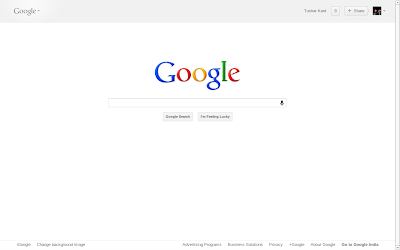The image captures a Google search page with a light gray background. The iconic Google logo is prominently displayed in the center, featuring a capital "G" in blue, followed by a lowercase "o" in red, another lowercase "o" in yellow, a lowercase "g" in blue, a lowercase "l" in green, and a lowercase "e" in red. Below the logo, there is the familiar search bar, accompanied by two buttons, whose labels are indistinguishable due to blurriness.

In the top right corner of the image, there are several clickable icons, although their details are too blurry to make out clearly. The last icon appears to be a profile picture set against a black background, depicting two individuals.

At the bottom of the image, there is a section with very small text links. On the left side, there are two clickable areas. Moving towards the center and stretching to the lower right corner, there are six additional clickable areas, neatly aligned in a row.